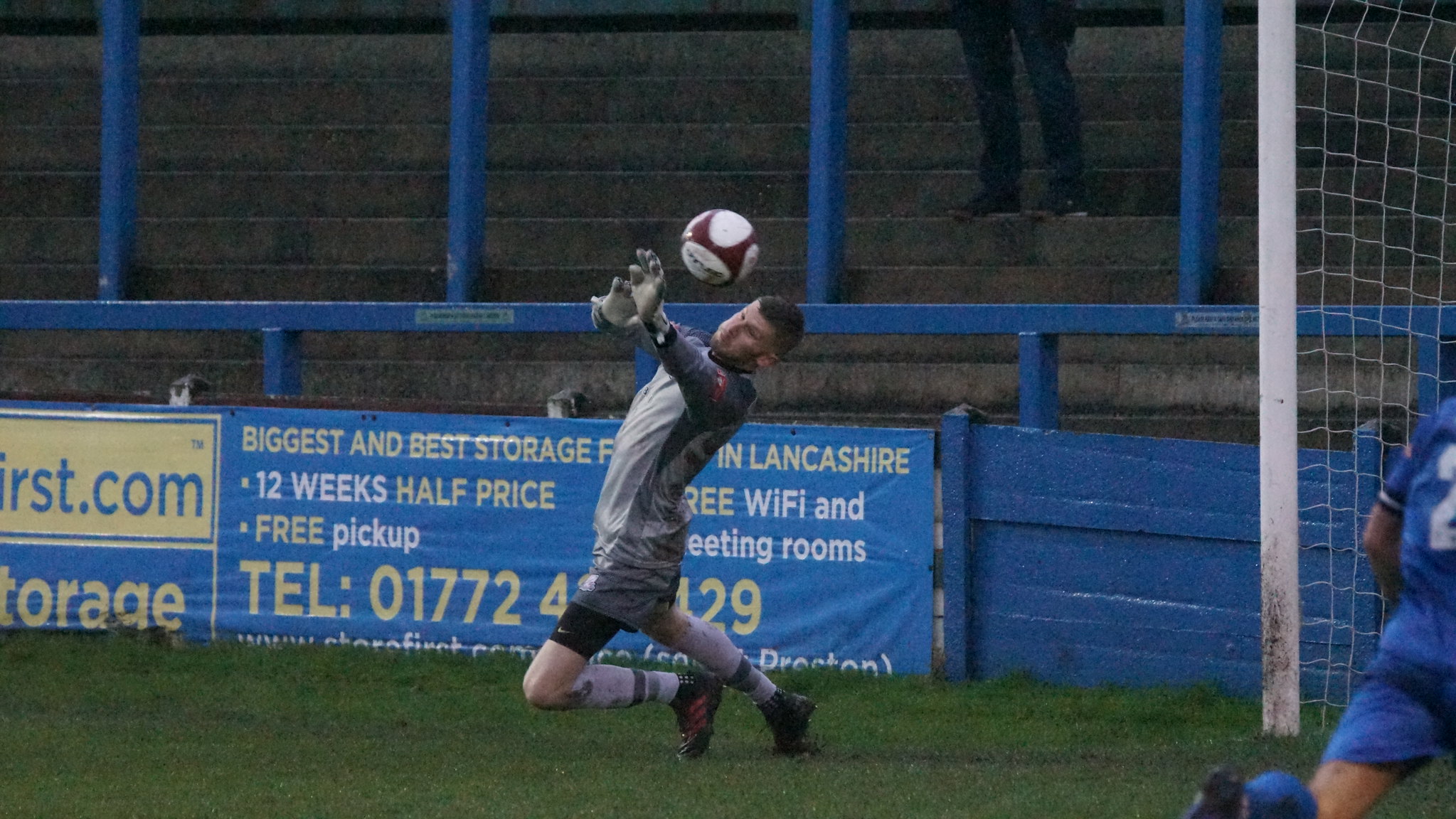This photograph captures an intense moment during a soccer match, focusing on a goalie wearing a grayish-silver uniform with gloves, black shoes featuring Adidas stripes, and little black spandex visible below his shorts adorned with red stripes. The goalie appears to be in the act of making a crucial save, with the soccer ball suspended in mid-air just above his head and his arms outstretched. In the lower right corner, there's a partially visible player in a royal blue uniform, captured in motion as he runs. The scene is framed by a blue fence surrounding the playing field, with stone steps serving as bleachers visible behind the fence. The edge of the goal, with its white pole and netting, appears on the right side of the photograph, adding context to the action unfolding on the field.